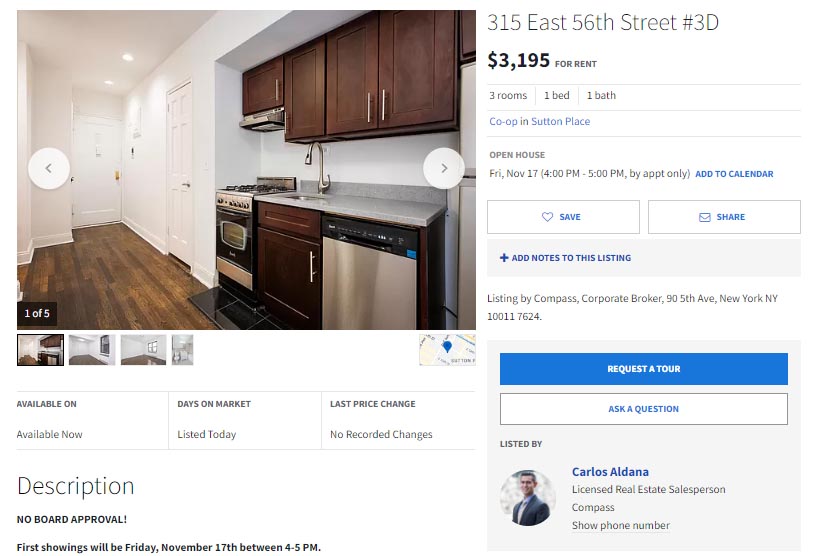The image displays a detailed listing for an apartment available for rent in a horizontal landscape format. In the top left section, there is a photo showcasing the interior of the apartment. The image features a short hallway with white walls, a white door at the end, and another white door on the right side. The flooring is brown wood, leading into the kitchen area. 

The kitchen is equipped with a black and silver stove and oven, a grayish countertop integrating a sink, and dark brown, almost mahogany-like cabinets both below and overhead. Additionally, there is a silver and black dishwasher under the counter and a large vent above the stove. A small section of black tiling is visible in front of the oven, enhancing the kitchen's aesthetic.

This is the first of five photos available in the listing. The details below the image indicate that the apartment is available now. The price is listed as $3,195 per month with no recorded changes, and it was listed today. The listing highlights that no board approval is required for renting. 

The first available showings are scheduled for Friday, November 17th, from 4:00 to 5:00 PM by appointment only. The apartment, located at 315 East 56th Street, number 3D, consists of three rooms including one bedroom and one bathroom. It is a co-op property. 

Additional options on the listing include the ability to add the open house to a calendar, save and share the listing, and add notes. This listing is provided by Compass Corporate Broker, situated at 95th Avenue, New York, New York, 10017-7624.